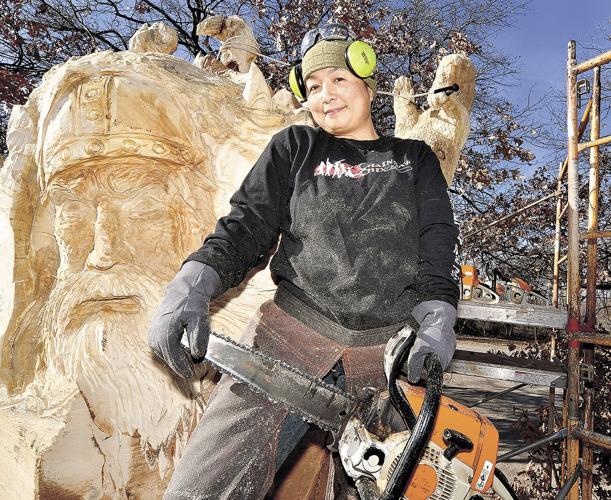In this detailed outdoor photograph taken during the daytime, we see a scene indicative of fall or early winter, depicted by the dead leaves and stark tree branches against a blue sky backdrop on the right-hand side. The focal point is a woman of Native American descent, positioned centrally and shown from the knees up. She is attired in a long-sleeve black sweater showcasing a red and white design featuring people, black pants, and gray-colored work gloves. Her outfit also includes leather protective chaps over blue jeans. 

On her head, she dons a green beanie topped with yellow ear protection, and a pair of transparent safety glasses rests on her forehead. She holds a chainsaw, characterized by an orange base and a silver chain, with one hand on the blade and the other on the handle. Her posture is dynamic, with one leg raised as she pulls the chainsaw towards it, and her face bears a slight smile, looking somewhat downward.

The scene is enriched with a scattering of sawdust around her, indicating recent woodwork activity. Behind her, there is a detailed wood carving of a man with a beard and a Viking helmet, adding an artistic element to the image. To the right, some scaffolding and shelves with additional chainsaws are visible, emphasizing the working environment. Overall, the image captures a lively moment of craftsmanship and nature intertwined.